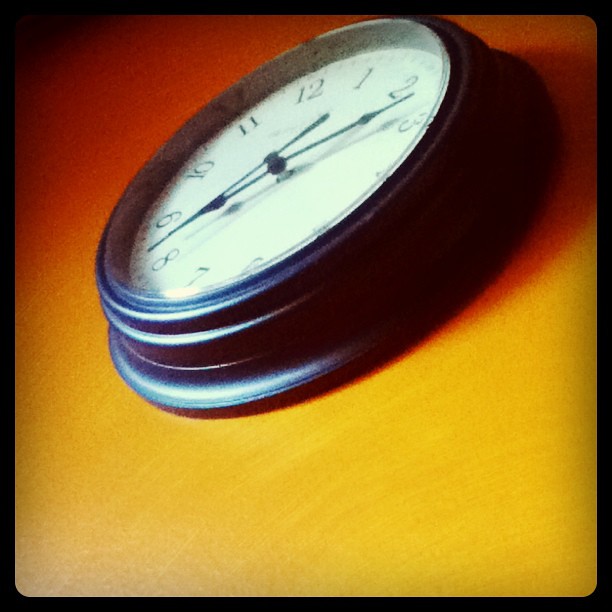The image captures a thick, circular clock taken from a downward left angle, mounted on a two-toned wall that transitions from white at the bottom to a red hue at the top. The clock's casing is predominantly black, featuring an intricate circular design along its border. The clock face, protected by a glass covering, is primarily white with black numbers and is marked by five small dashes between each numeral. The hour hand is positioned between the numbers 8 and 9, while the minute hand lies between 2 and 3, both hands being black with a spade shape towards their ends. The lighting comes from the bottom left, casting a shadow that extends up and to the right. The clock appears slightly raised from the wall due to the lip around its edge. The image is of low resolution and set within a square frame, with the wall exhibiting a blend of yellow and red colors.